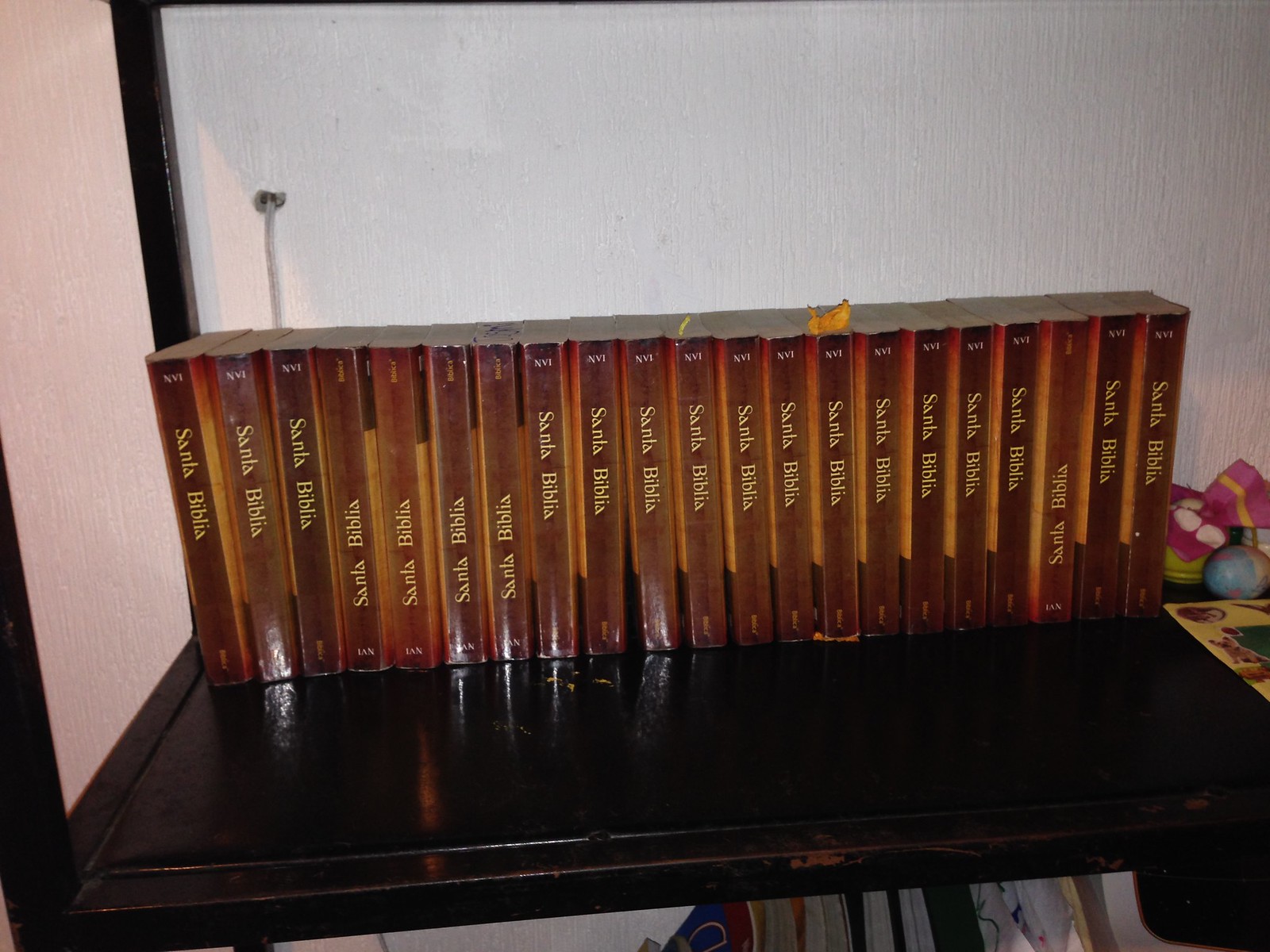This photo captures a section of a black bookshelf at chest level, lined with around 20 brown paperback Bibles. The spines of these books, uniformly displaying the yellow text "Santa Biblia," create a cohesive visual pattern. However, the neat arrangement is disrupted by five upside-down volumes, specifically the 4th through 7th and 19th books from the left, which break the otherwise consistent alignment. The setting appears to be a bedroom, adding a personal touch to this organized collection.